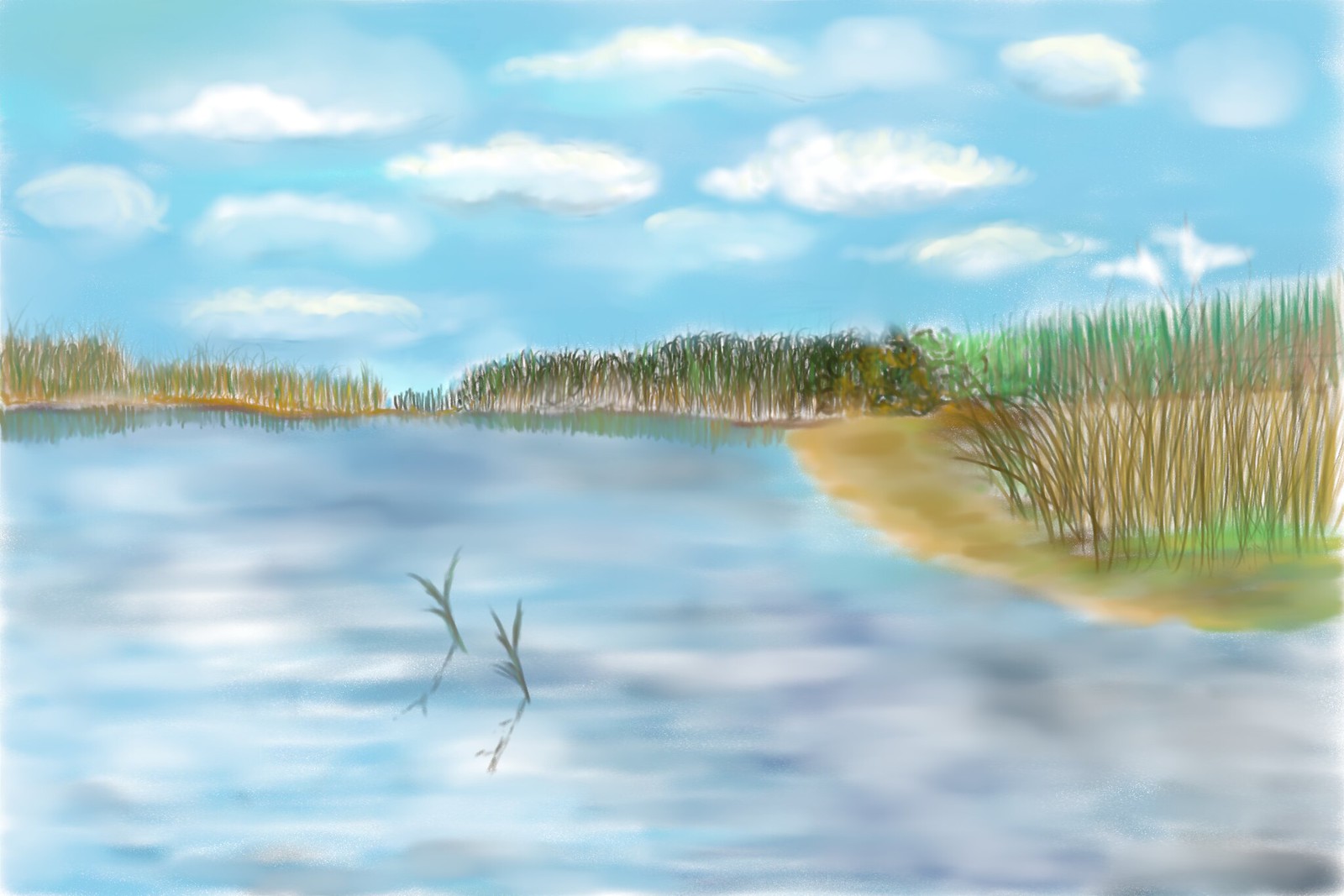This illustration, likely a watercolor or color pencil piece, depicts a tranquil river scene in the foreground, extending across most of the image. On the right side of the river, a small shoreline hosts reeds or Spartina grass, giving it a marsh-like appearance. The horizon features more dense grassy areas, both to the right and left, enhancing the scenery's natural feel. Two sticks or pieces of aquatic plants protrude from the water near the center-left, adding to the scene's realism. The sky above is a vibrant blue, adorned with fluffy white clouds, which the water below mirrors perfectly, creating a serene and reflective ambiance.